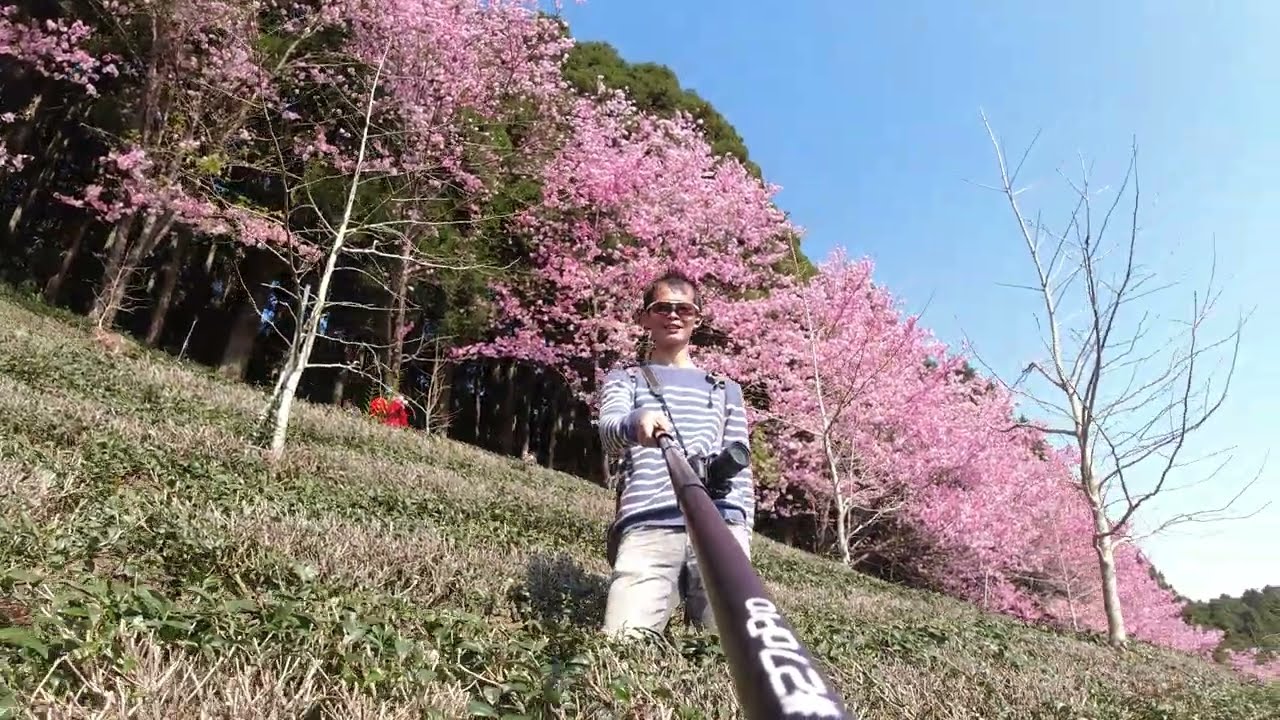In this image, a man with short black spiky hair and wearing sunglasses is kneeling on the grass, taking a selfie with a long black selfie stick that has white text reading #270 Pro on it. He is dressed in a long-sleeved blue shirt with white stripes and white pants. Around his neck hangs a large black camera with a substantial lens, indicating a professional interest in photography. The setting appears to be early spring, as evidenced by the cherry blossom trees in full bloom behind him, contrasting with other trees that are still bare. The clear blue sky and the lush greenery of the area add to the vibrant and refreshing ambiance of the scene.